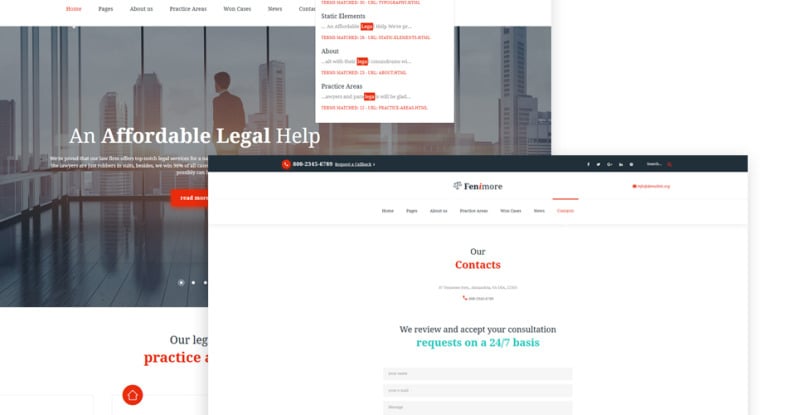In the foreground, a semi-transparent web page partially overlays another web page in the background. The background image is a full-page photograph depicting a sophisticated corporate corner office with floor-to-ceiling windows. A man dressed in a suit and a white shirt, with his hands in his pockets, gazes out at a cityscape filled with numerous skyscrapers, characterized by a misty, gray ambiance suggestive of a cloudy morning. 

Superimposed on this background image, white text reads "An Affordable Legal Help." Above this, the website's navigation menu displays options labeled: Home, Pages, About Us, Practice Areas, an unreadable option, News, and another unreadable option. One of these options features a drop-down menu containing text in black and red on a white background, although the specific word is not legible.

The overlaying page includes a thin black ribbon across its top. Its main background is white and prominently features "Fenimore" in blue, with the 'I' colored red, adjacent to a logo. Below this heading, small unreadable text is present, followed by the bold red word "Contacts," and additional content further down the page.